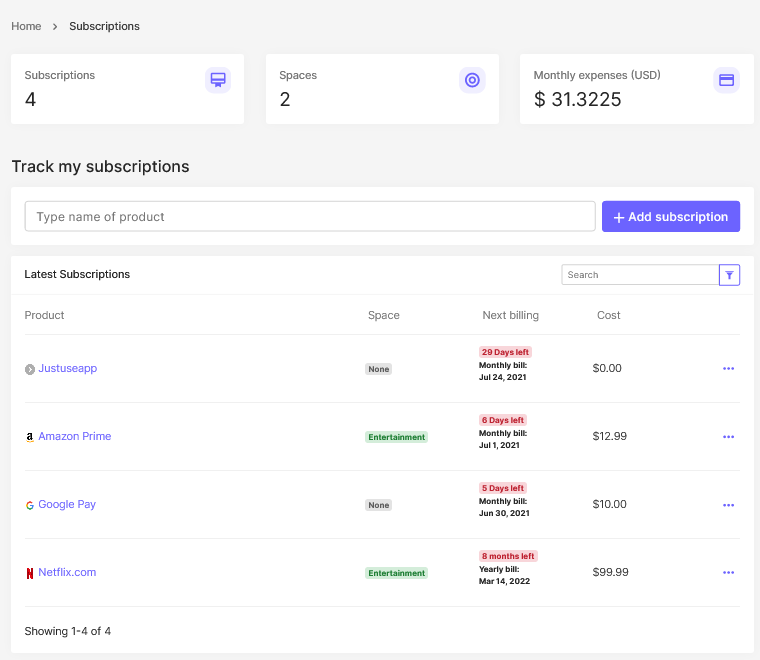The image appears to be a screenshot from a subscription management app designed to track and organize various subscription services. Dominated by a large, primarily white square background with subtle accents of light blue at the top, the screenshot presents a well-structured layout.

In the top-left corner, a navigation header displays "Home" with a small arrow pointing to the right, followed by "Subscriptions". Beneath this header, on a white rectangular background, it reads “Subscriptions for”, and to its right, “Spaces to”. Adjacent to this, it lists "Monthly expenses (USD): $31.3225".

The main body of the image features a search bar labeled “Type name of product for searching”. Below this bar is a section titled "Latest Subscriptions", with columns labeled "Product", "Space", "Next Billing", and "Cost".

The detailed list of subscriptions includes:
1. **Just Use App**
   - Space: None
   - Next Billing: 29 days left, monthly bill on July 24th, 2021
   - Cost: $0

2. **Amazon Prime (Entertainment)**
   - Space: None
   - Next Billing: 6 days left, monthly bill on July 1st, 2021
   - Cost: $12.99

3. **Google Pay**
   - Space: None
   - Next Billing: 5 days left, monthly bill on June 30th, 2021
   - Cost: $10

4. **Netflix.com (Entertainment)**
   - Space: None
   - Next Billing: 8 months left, yearly bill on March 14th, 2022
   - Cost: $99.99

In the bottom left-hand corner, it indicates “Showing 1 of 4”, suggesting pagination with this view representing the first page.

Overall, the screenshot showcases a subscription monitoring service, providing users with a streamlined overview of their active subscriptions, associated costs, and upcoming billing dates.